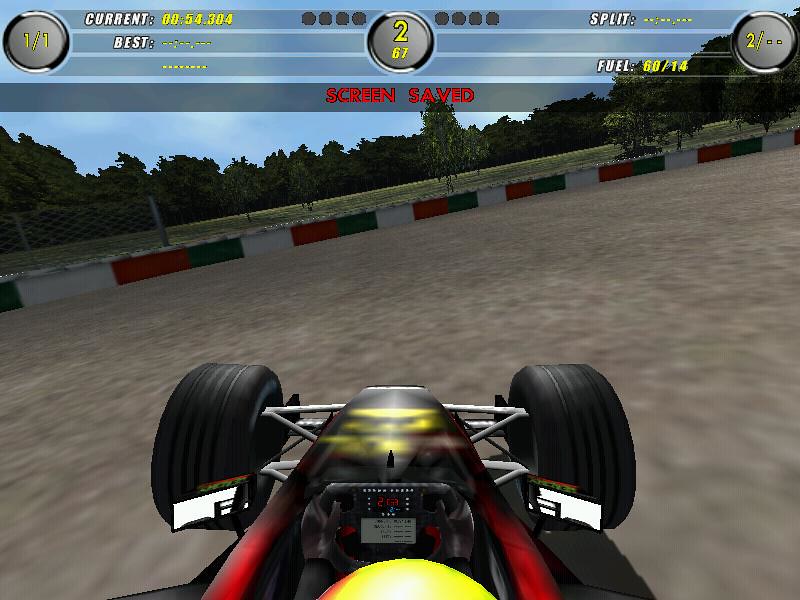High-resolution screenshot from a modern racing video game, exhibiting vivid, lifelike graphics that sit between an illustration and film. The image features a Formula One-type car or similar racing vehicle, captured from a rear angle on an outdoor track. The sleek racing car, primarily red and black with a hint of yellow from the driver's helmet, is set against a slightly tilted brown track. Above the scene, a clear blue sky and scattered trees suggest it's an open-air circuit. The on-screen display shows various metrics like 'current', 'best', 'split', 'fuel' and a curious circle marked "2/67", indicating perhaps lap numbers or positions.